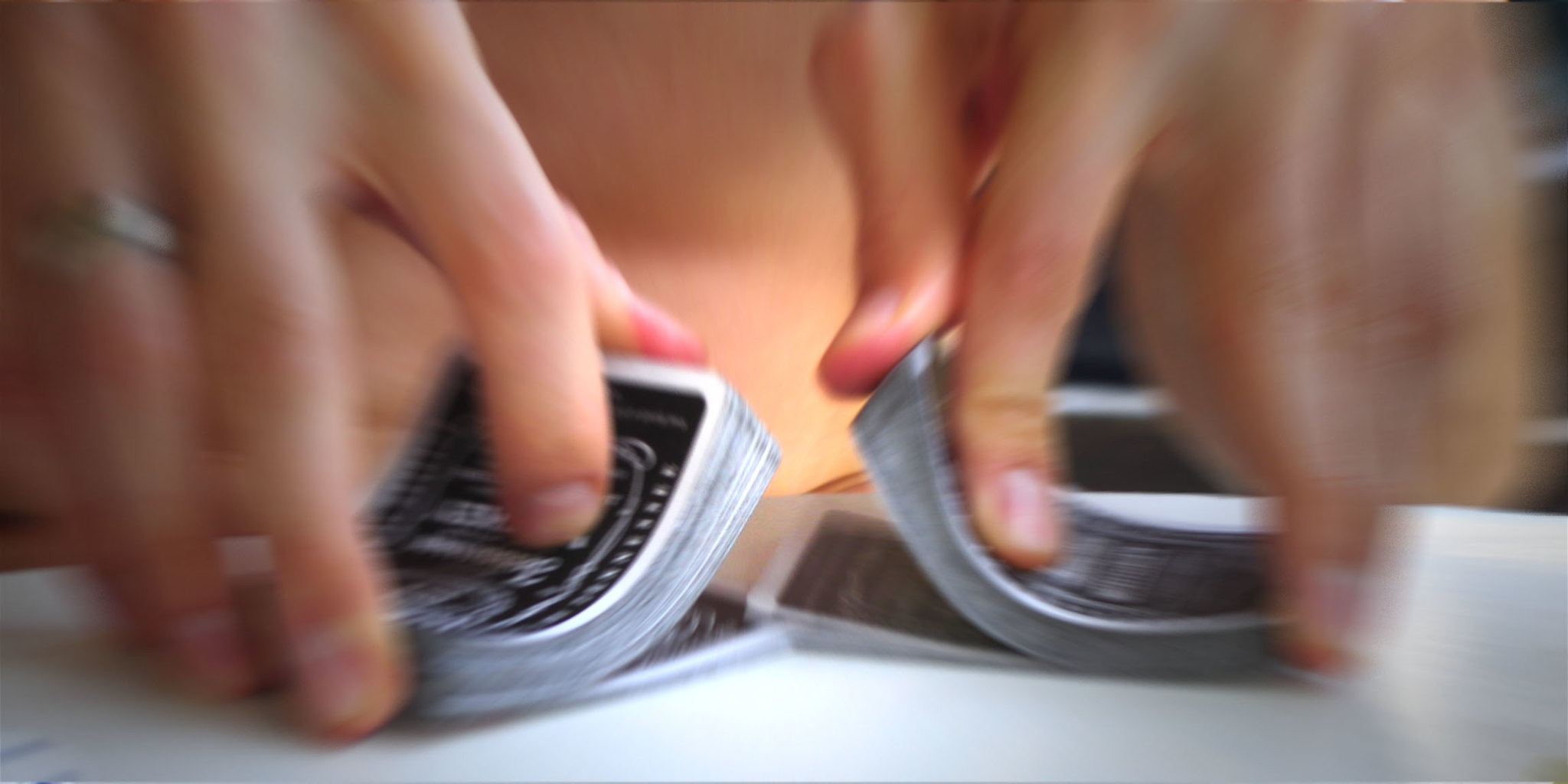A close-up photograph captures the dynamic moment of someone shuffling a deck of cards on a white table. The image is primarily focused on the center where the shuffling action occurs, revealing the individual's index fingers and thumbs bending two halves of the deck upward as they prepare to blend them together. The cards, which are black with elegant white designs on their backs, form the central focal point of the composition.

The blurriness increases towards the edges of the photo, particularly around the person's hands, which are descending from the upper corners— the right hand on the left side of the image and the left hand on the right side. The motion of shuffling is suggested by the extreme blurriness of the hands and parts of the deck.

In the background, there is an indistinct, skin-toned blur that fills the space behind the table, which might be a person, a wall, or even a piece of wood, though its true identity is obscured by the lack of focus. Additionally, on the upper right side of the image, there is a dark brown wall featuring horizontal white lines stretching from the center to the right.

The overall scene portrays the action-packed motion of shuffling playing cards, with the photograph emphasizing the speed and dexterity involved in the activity.